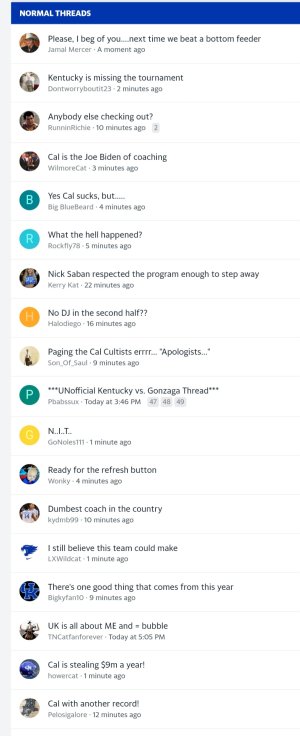The image is a tall screenshot featuring a structured layout. At the top, there's a header bar in blue with white text that reads "Normal Threads." Below this, the content area has a plain white background, arranged in rows. There are 18 individual comments visible, each initiated by a colorful, round avatar image or photograph. Each row comprises a dark text header, the name of the person who left the comment, and a timestamp indicating when the comment was posted. The details and order create a clear, informative, and visually organized display of the threads.